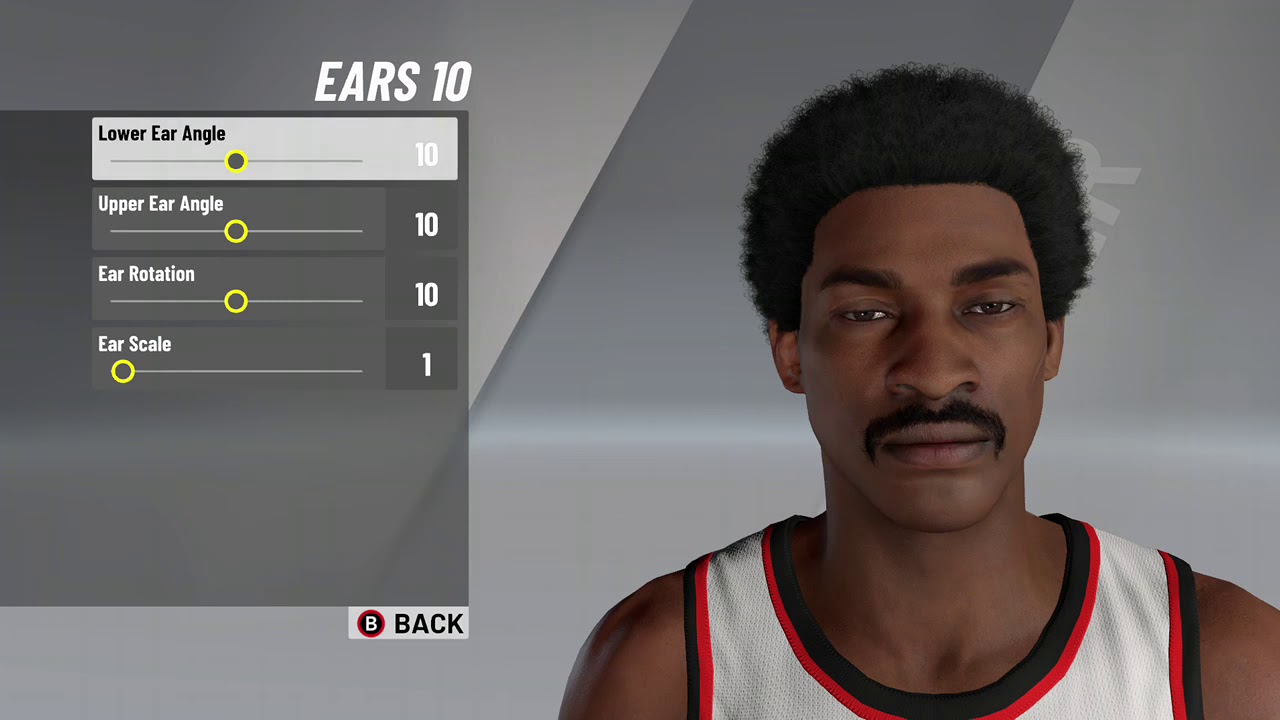The image captures a scene from a video or computer game, featuring a character customization screen. On the left side of the image, there's an African American man with dark skin and a distinctive appearance. He has a black afro, thick black eyebrows, and slightly hooded, droopy eyelids that reveal his brown eyes. His facial features also include a black mustache and a wide-set nose. He is dressed in a stylish, mesh basketball jersey colored in white, red, and black. 

The background behind the character is a gradient of gray, with sections of lighter and darker shades, including a notable darker gray strip visible behind his head. To one side of his head, white letters are partially visible, while on the other side, a gray box displays customization options for his facial features.

This gray box includes several descriptors in white text indicating various ear adjustments: “ears 10,” “lower ear angle 10,” “upper ear angle 10,” “ear rotation 10,” and “ear scale 1.” Each adjustment option is followed by a gray circle with a yellow outline. Below this, an off-white box labeled “back” in black text is visible. To the right of this label, there’s a red and black circle featuring a prominent white “B.” 

The image quality is exceptionally clear and crisp, making all text and visual elements easy to read and distinguish.